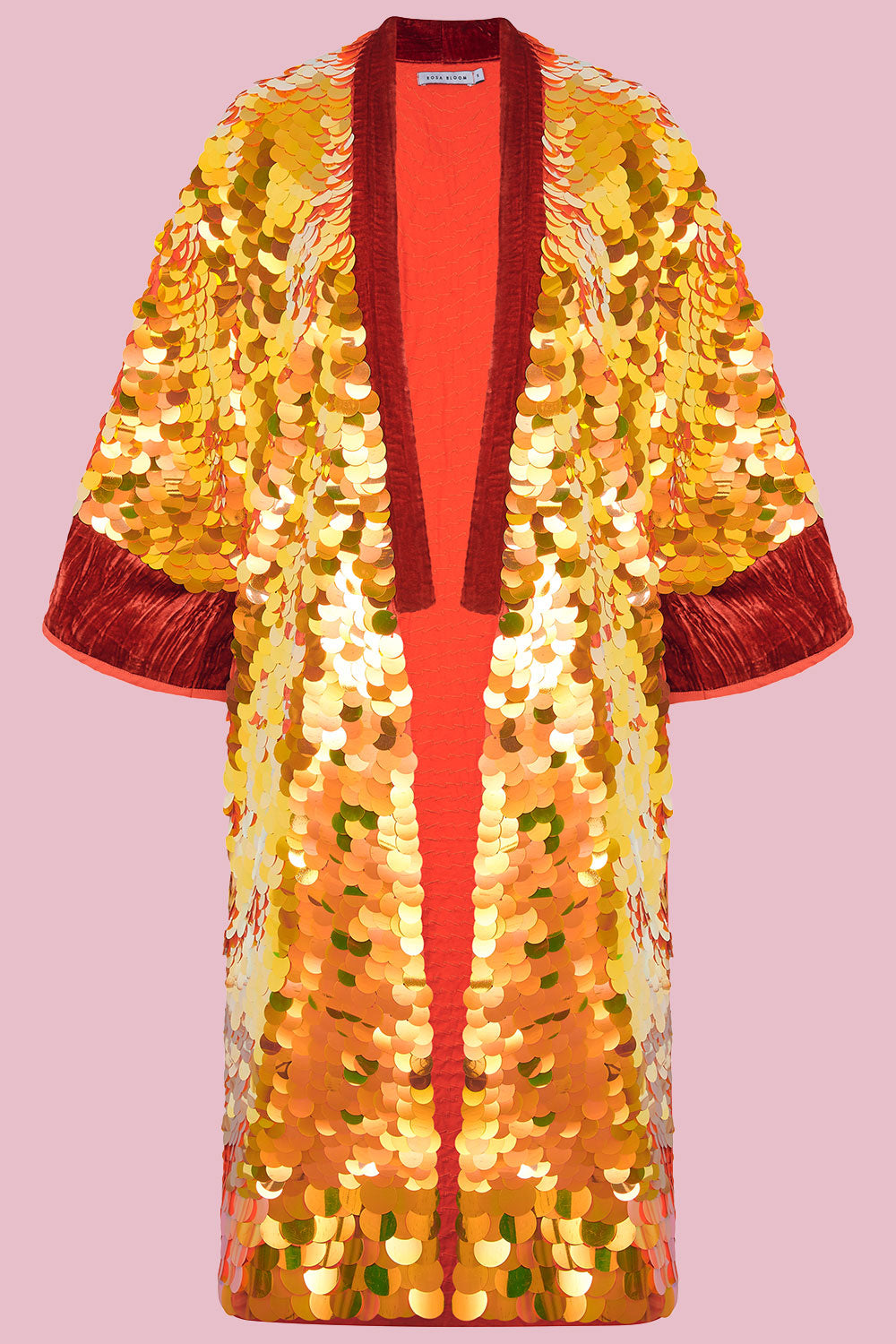This image showcases an intricately designed robe, heavily embellished with large, gold, reflective sequins that give it a scale-like appearance. The robe features brushed velvet seams in a vivid red hue around the neckline and sleeves, which extend to about the elbow. The interior is similarly red, presenting a tiered layout. Set against a pink backdrop, the floor-length garment hangs open without any fastenings, resembling both a luxurious housecoat and a kimono. The dazzling sequins and shimmering fabrics create a striking, opulent effect, making the robe a standout piece either as a product photograph or a museum exhibit.